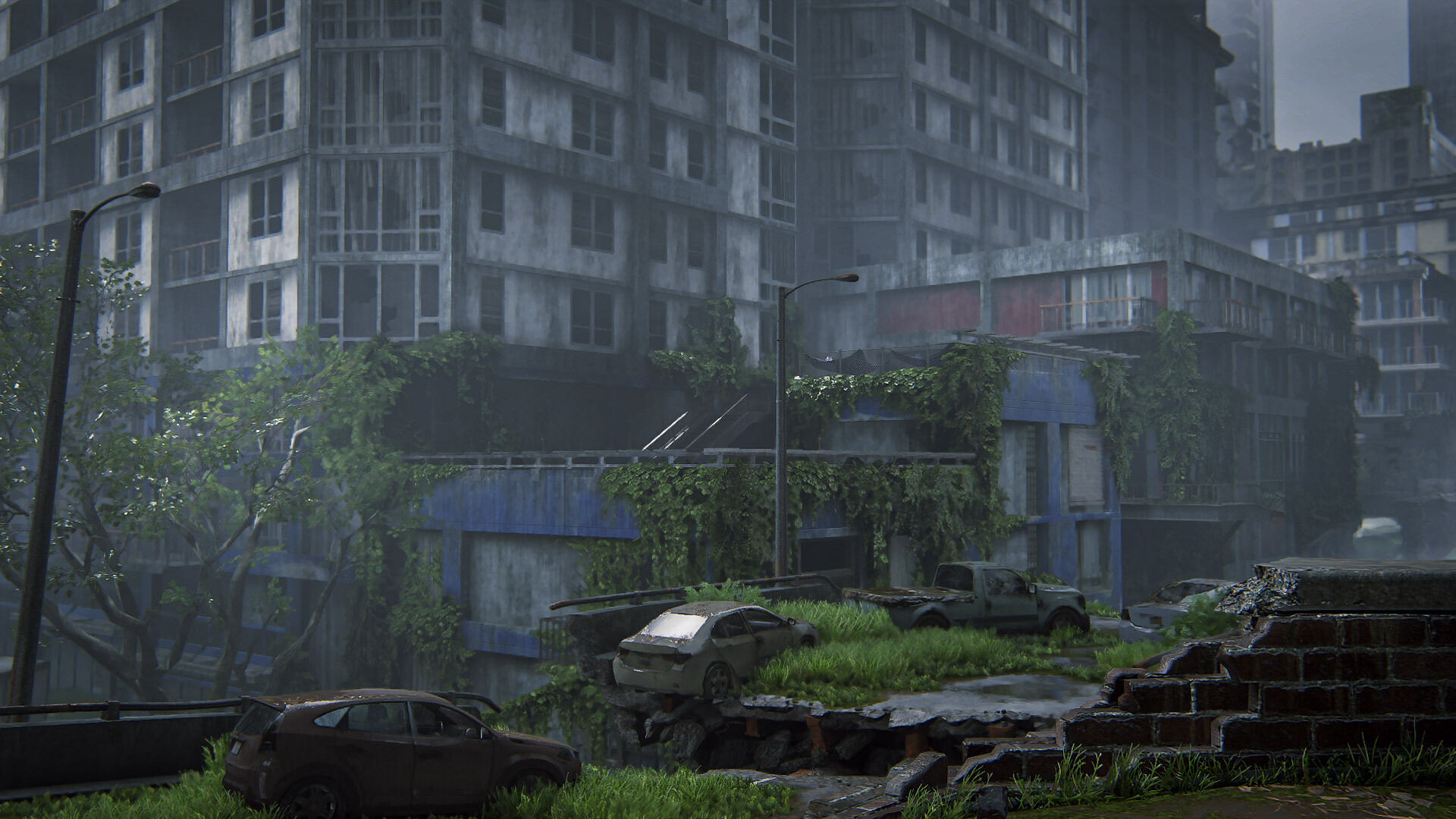The image portrays a haunting post-apocalyptic scene of an abandoned city shrouded under a dark, cloudy sky. The skyline is filled with decrepit, broken skyscrapers, their facades marred by time and neglect, now overgrown with vines and vegetation. In the forefront, a collapsed bridge juts out dramatically, its roadway fragmented into a chasm. Three abandoned cars are scattered precariously—some teetering on the edges of the broken structures, one even hanging off a cliff-like ledge of the bridge. The stone walls and roadways are half fallen apart, covered in grass and greenery, emphasizing the eerie silence and desolation. The atmosphere is exceptionally dreary and spooky, painting a vivid picture of a world long forsaken by its inhabitants.